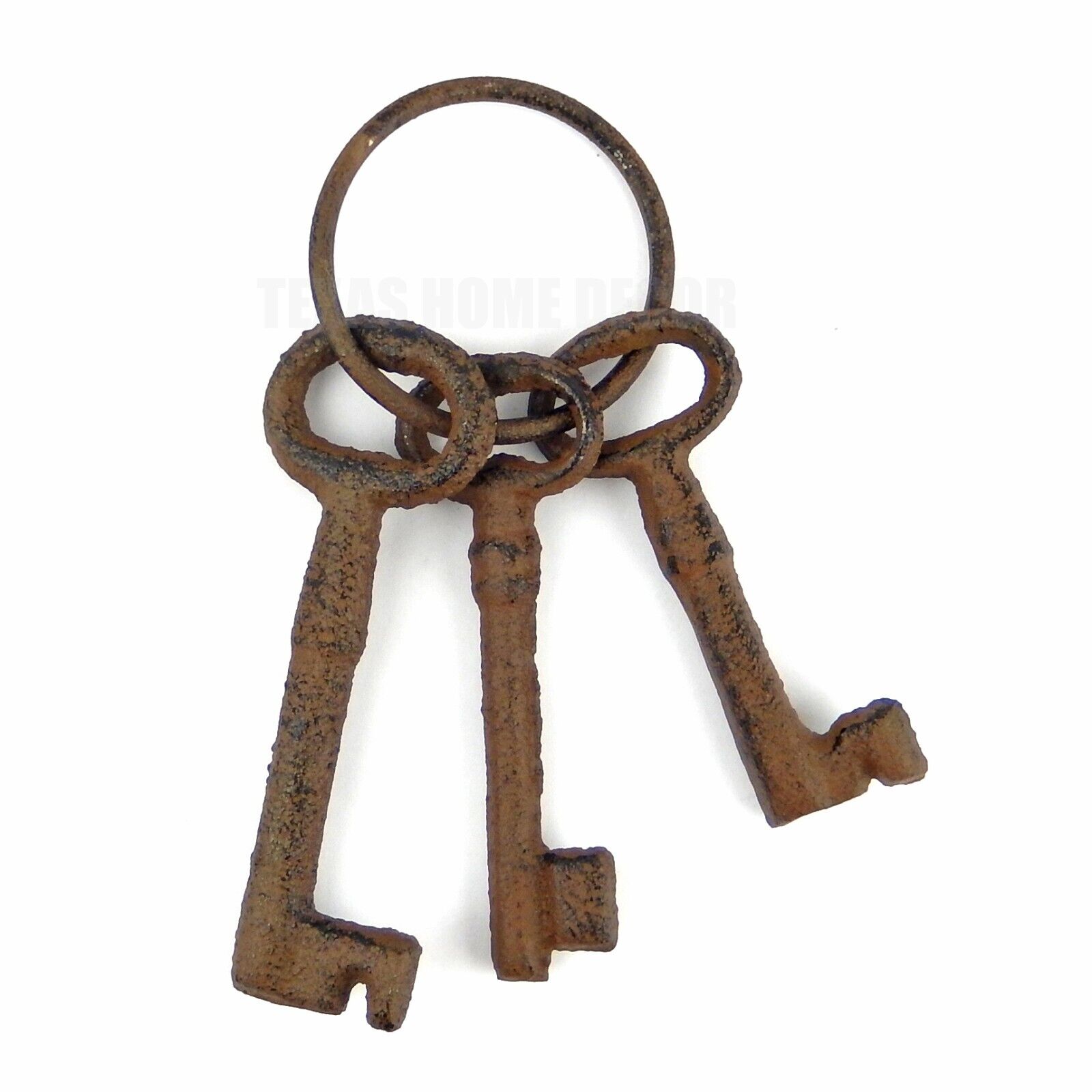In this detailed image against a white background, there is a round piece of metal heavily coated in rust, functioning as a large ring holding three ancient, cast iron keys. These keys resemble jailer or skeleton keys, characterized by their looped tops, long shafts, and intricate, curved ends that would fit into sizable locks. Each key varies slightly in size, with the largest on the left, a smaller one in the middle, and the smallest on the right. Despite their antiqued and rusted appearance, the keys still display hints of their original coppery gold sheen. The overall look of these keys suggests they have a historical or decorative purpose, possibly as part of a museum exhibition of ancient artifacts.